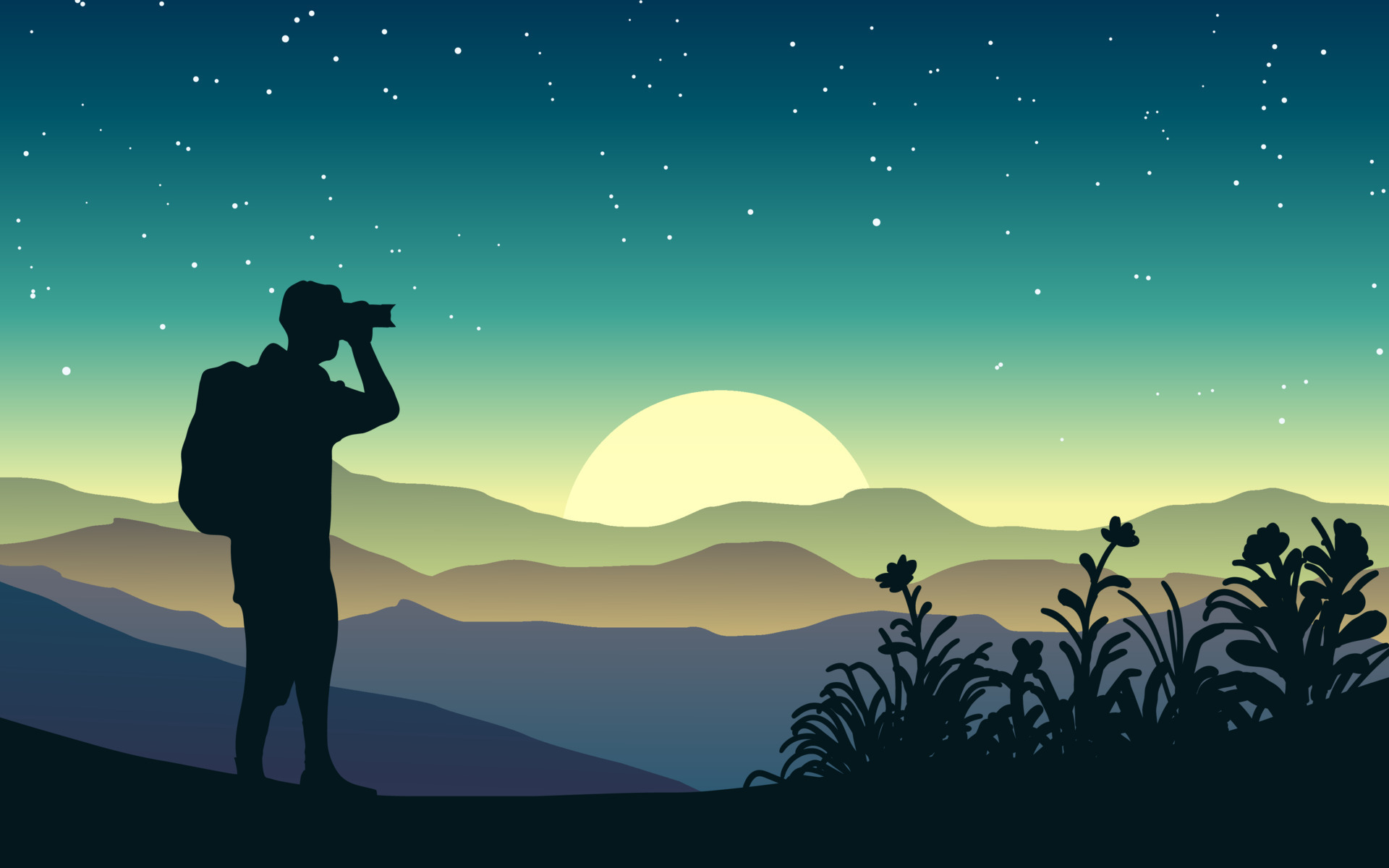The computer-generated image depicts a silhouetted man standing in the foreground on a dark surface, possibly hiking or camping. The man, outlined in a very dark blue, wears a large backpack or daypack and holds binoculars up to his eyes, gazing into the clear, starry night sky. To his right, dark silhouetted plants and flowers grow. Behind him, the landscape features a series of mountain ranges in progressively lighter and muted shades of indigo, blue, tan, and yellow-green. A setting sun, halfway visible, casts a faint glow, highlighting the mountains. The simplicity of the drawing emphasizes the serene and contemplative atmosphere of this nighttime or sunset scene.